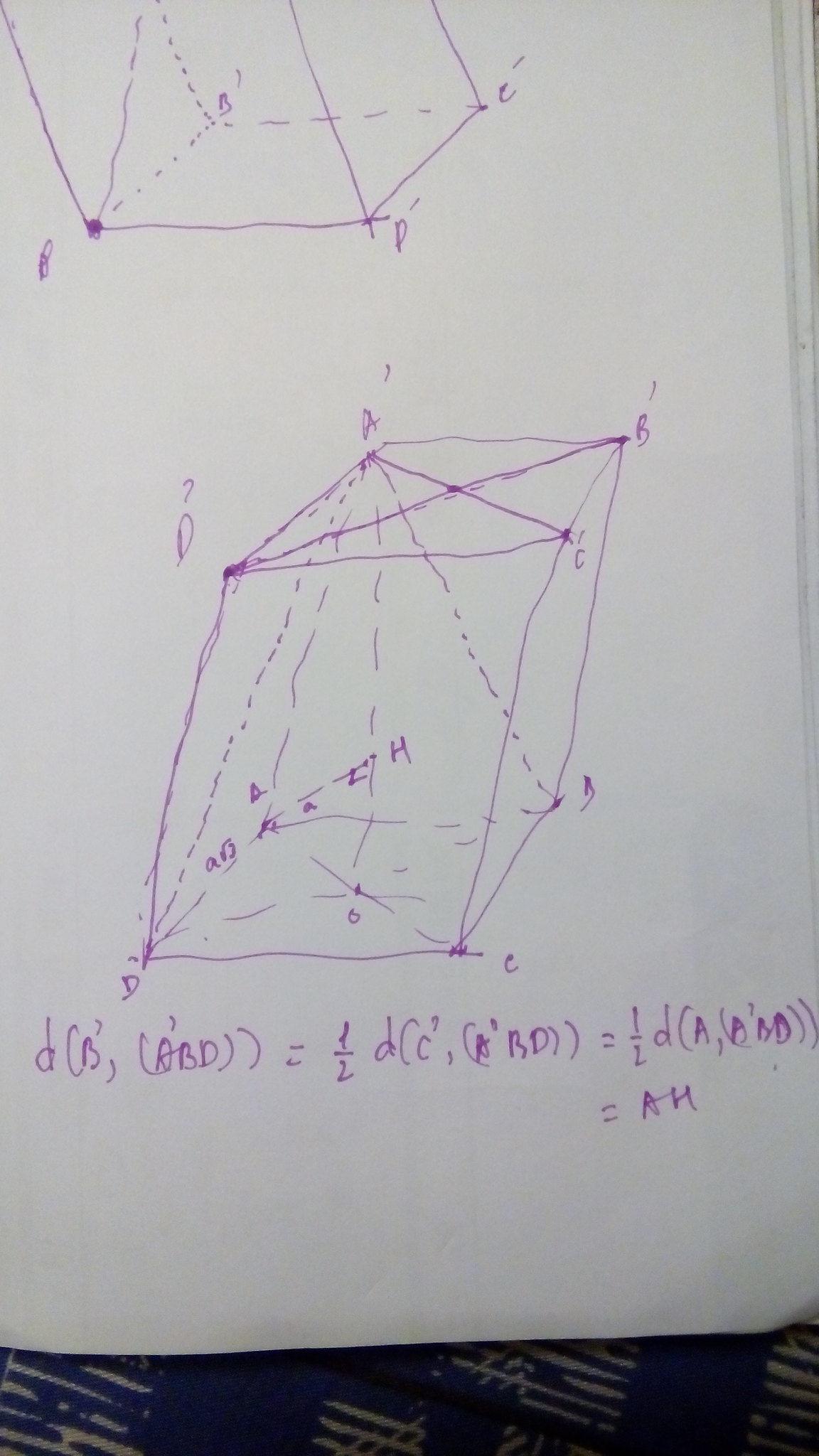This photograph depicts part of a white sheet of paper set against a background of blue fabric adorned with short, white and tan sketch-like stripes at the bottom edge. The paper features purplish handwritten content. Towards the upper left side, there is an outline of a cube, with each vertex labeled with a letter. Centrally located on the paper is a fully drawn cube, showing letters at each of its corners: 'A' at the back left, 'B' at the back right, 'D' at the front left, and 'C' at the front right. The cube's bottom vertices also exhibit corresponding labels. Below this depiction is a series of letters forming a large mathematical equation.